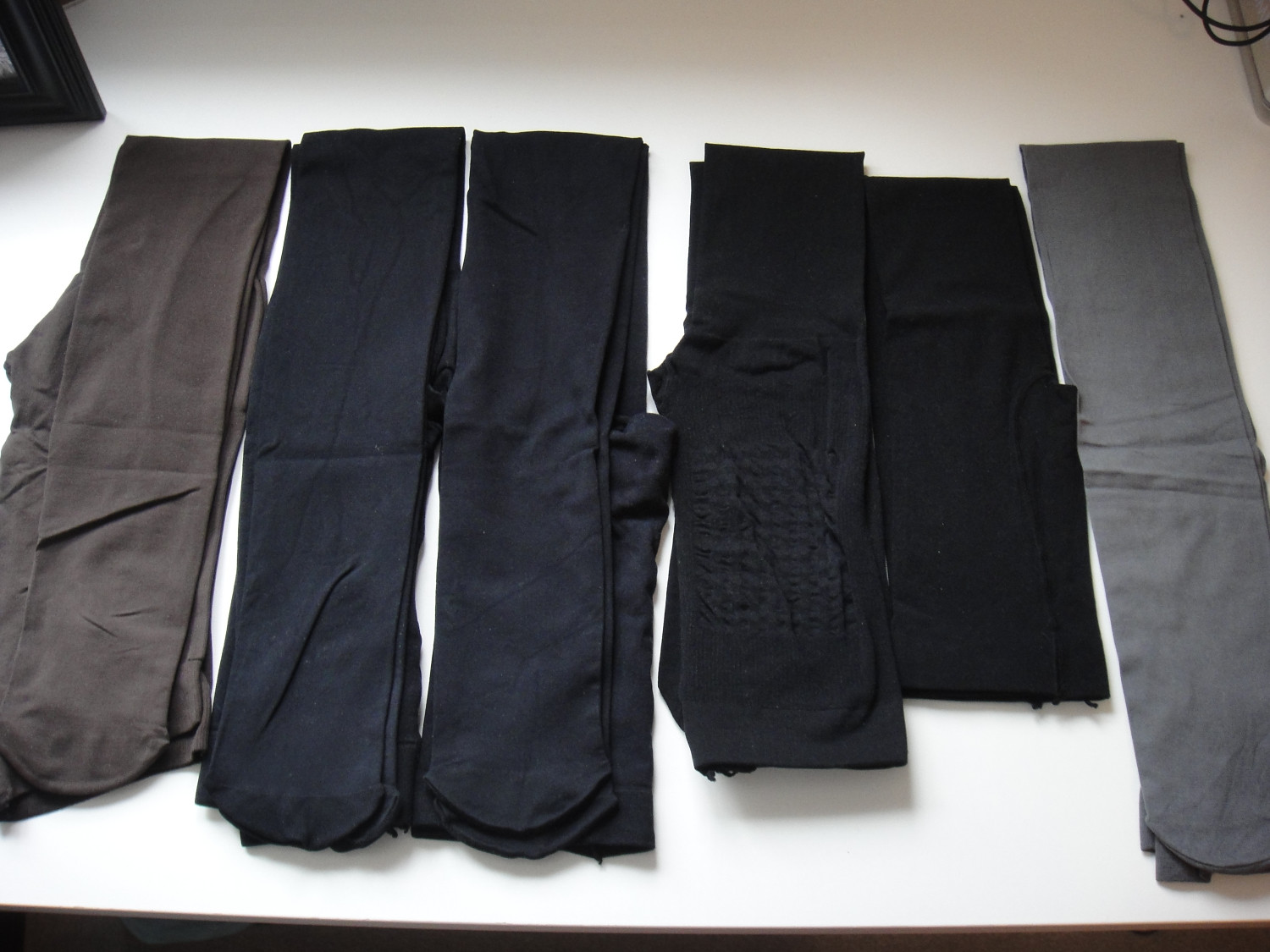The image captures a top-down view of six neatly folded pairs of pants arranged horizontally on a plain white background, possibly a table or countertop. From left to right, the pants display a gradient of colors: the first pair is a gray-brown, followed by two pairs of indigo-blue denim, the third of which has a slight purple tint. Next, there are two black pairs, with the fifth pair being a richer black, and finally, a gray pair that transitions from dark gray at the top to light gray at the bottom. A prominent crease marks the center of each pair, and the fourth pair exhibits a noticeable light gray imprint, suggesting it might have been scorched by an iron. The bottoms of the pants legs are all aligned at the bottom of the image, creating a visually organized display.